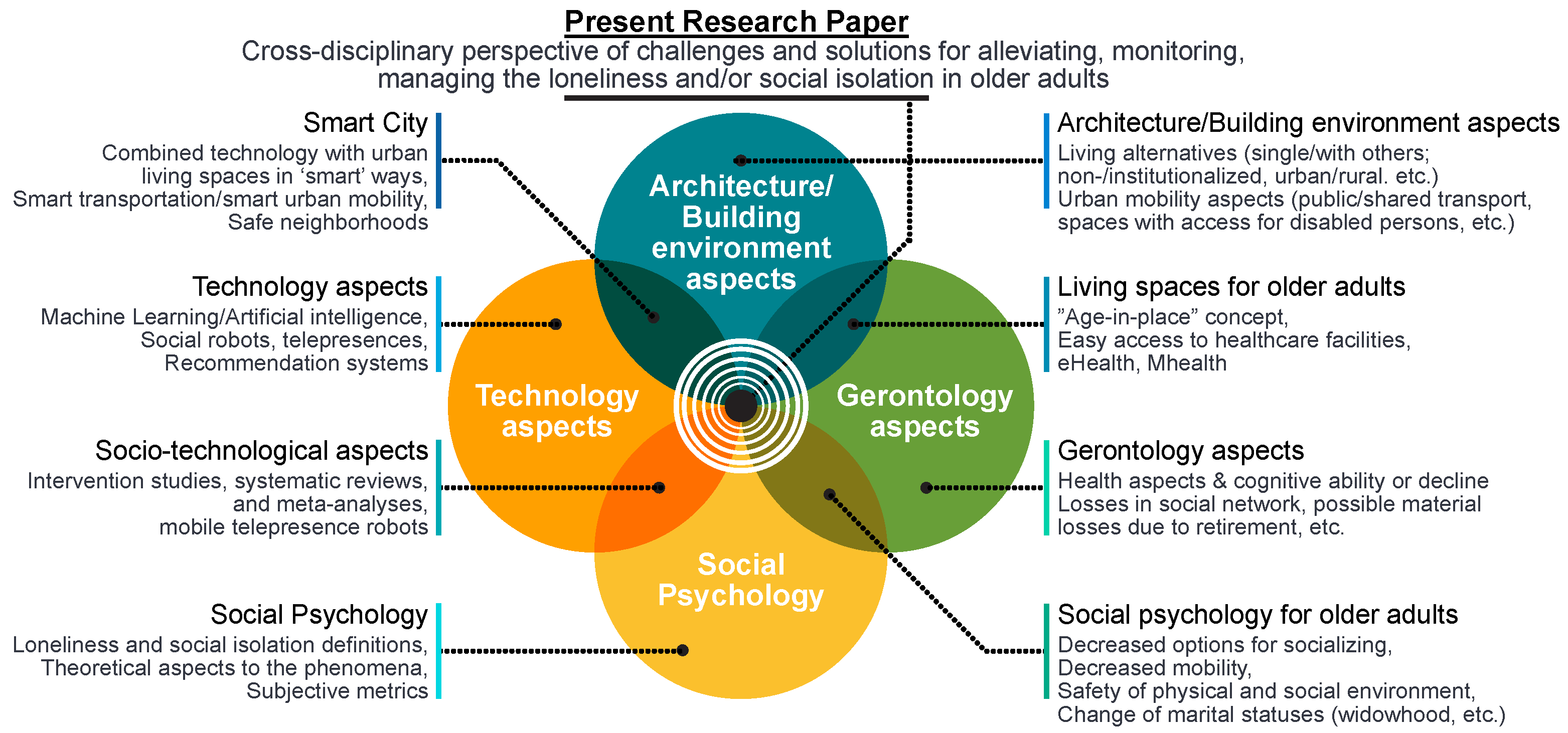The image is a detailed circular chart from an academic paper, titled "Present Research Paper: Cross-Disciplinary Perspective of Challenges and Solutions for Alleviating, Monitoring, Managing the Loneliness and/or Social Isolation in Older Adults." The core section of the diagram features four overlapping circles, each representing a distinct aspect: the blue circle for architecture and building environment aspects, the green circle for gerontology aspects, the yellow circle for social psychology, and the orange circle for technology aspects.

Surrounding these core circles are further detailed categories connected by lines, illustrating the intertwined nature of the disciplines. For example, the overlap between environment and technology highlights smart city aspects like smart transportation and safe neighborhoods. The overlap between technology and social psychology delves into socio-technological aspects such as machine learning, artificial intelligence, social robots, and recommendation systems. The intersection of social psychology and gerontology touches upon social psychological strategies for older adults, while the juncture of environment and gerontology explores improving living spaces for older adults.

This comprehensive diagram encapsulates the multifaceted challenges and integrated solutions for addressing loneliness and social isolation in older adults through a cross-disciplinary lens.